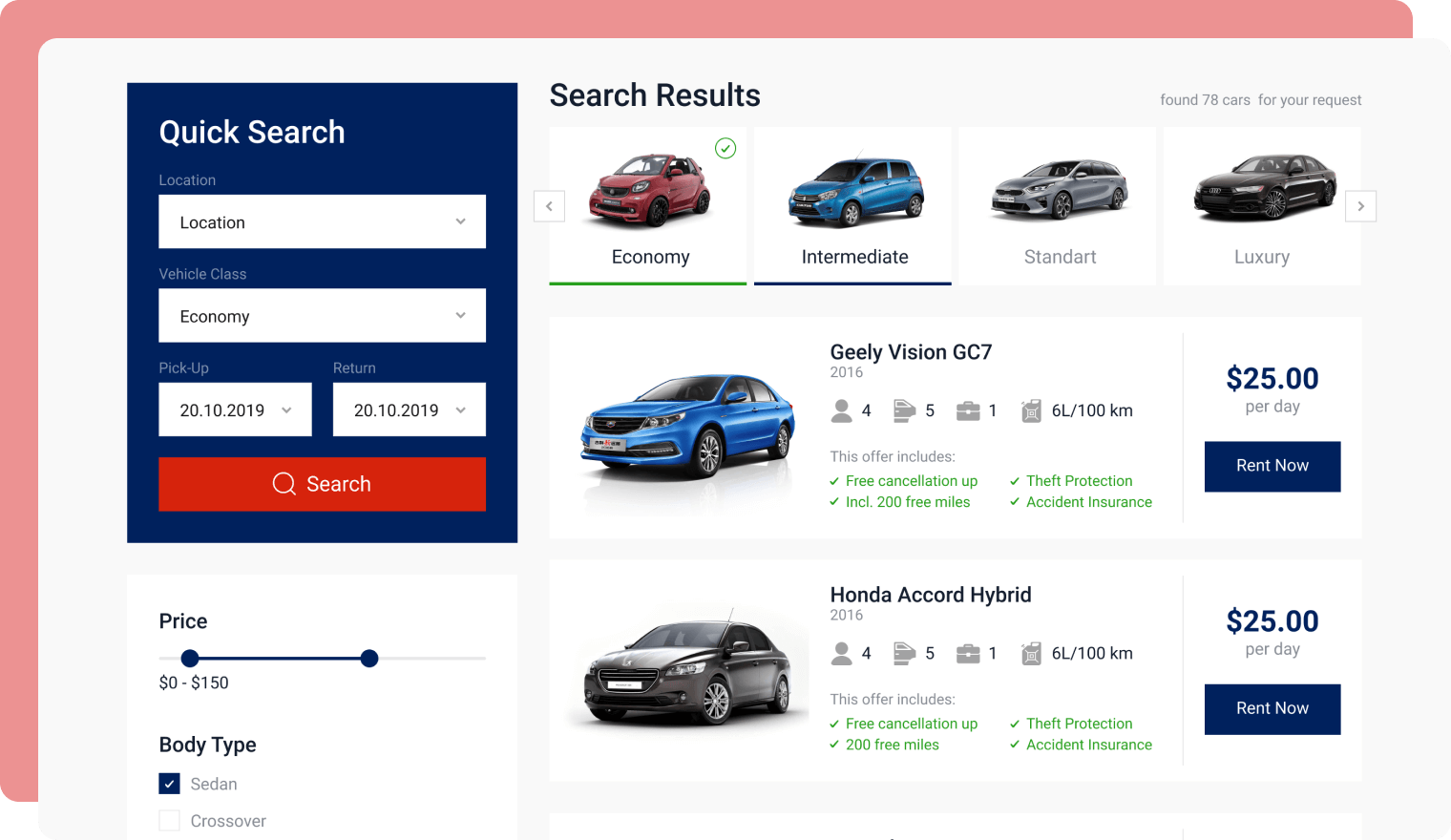Screenshot of a car rental website displaying various options and search results. On the left-hand side, there's a pink border surrounding a grayish box. Within it, a blue vertical box titled "Quick Search" allows users to choose rental preferences. The drop-down menus offer selections for location, car category, and pickup and return dates, both currently set to 20.10.2019. Below these options, a prominent red horizontal button labeled "Search" is visible. Further down, a white box offers a price range filter set from $0 to $150 and a "Body Type" filter, with the sedan option currently checked.

On the right-hand side, the search results indicate that 78 cars match the user’s criteria. At the top of the results section, four categories are available: Economy (currently selected), Intermediate, Standard, and Luxury. Each category displays different vehicle choices.

In the search results, two specific cars are shown. The first is a blue Geely Vision GC7, available for $25 per day, seating four people, and having five doors. Below it is a gray 2016 Honda Accord Hybrid, also priced at $25 per day and seats four people.